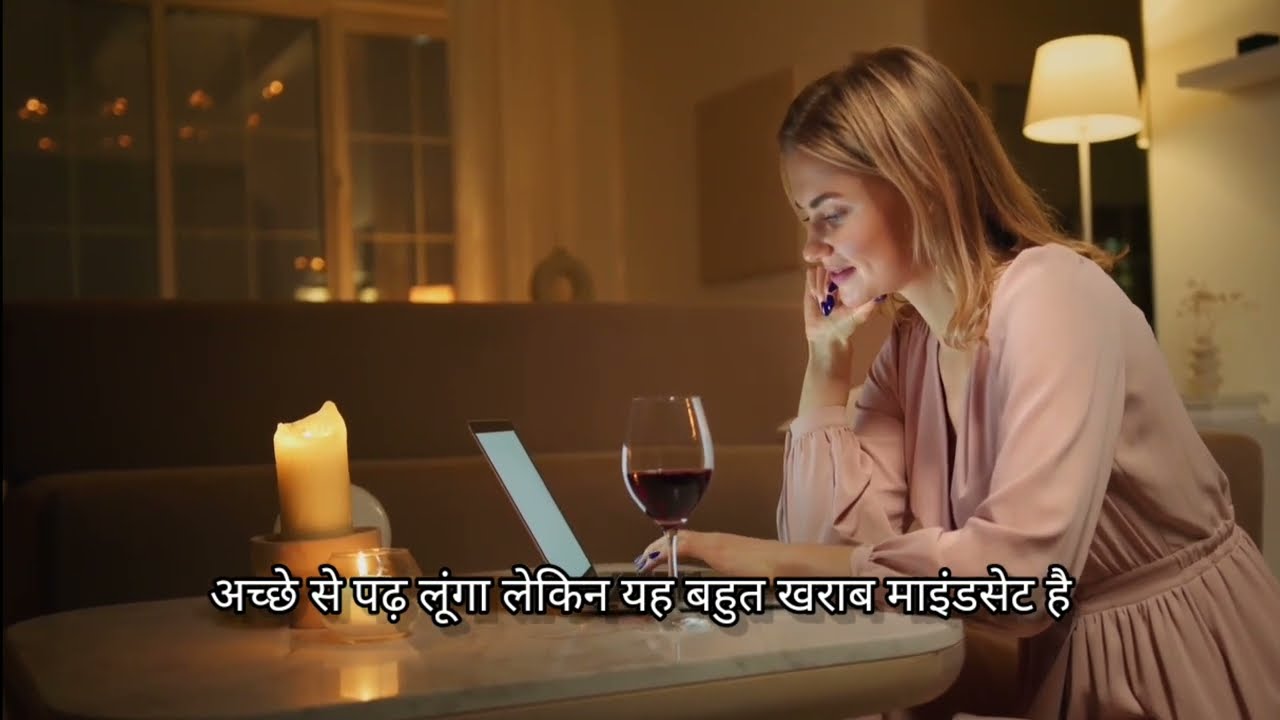In a cozy living room setting, a blonde-haired Caucasian woman with black painted nails is bent over a gray, thin laptop placed on a table, her fingers tapping away at the keyboard. Dressed elegantly in a pink dress, she appears focused on her screen. On the same table beside her hand sits a wine glass filled with a deep purple liquid, and two lit candles flicker in the center, adding a warm glow to the scene. 

The room's ambiance is enhanced by a tan-colored couch facing away from the table, a lamp anchored on a side table next to a lush green plant, and a hallway leading to another part of the house visible in the background. The table has a white marble countertop, contributing to the sophisticated atmosphere. Overall, her setting suggests a blend of work and leisure, creating an inviting atmosphere that could easily be part of a commercial or advertisement, possibly hinting at a luxurious, relaxing lifestyle.